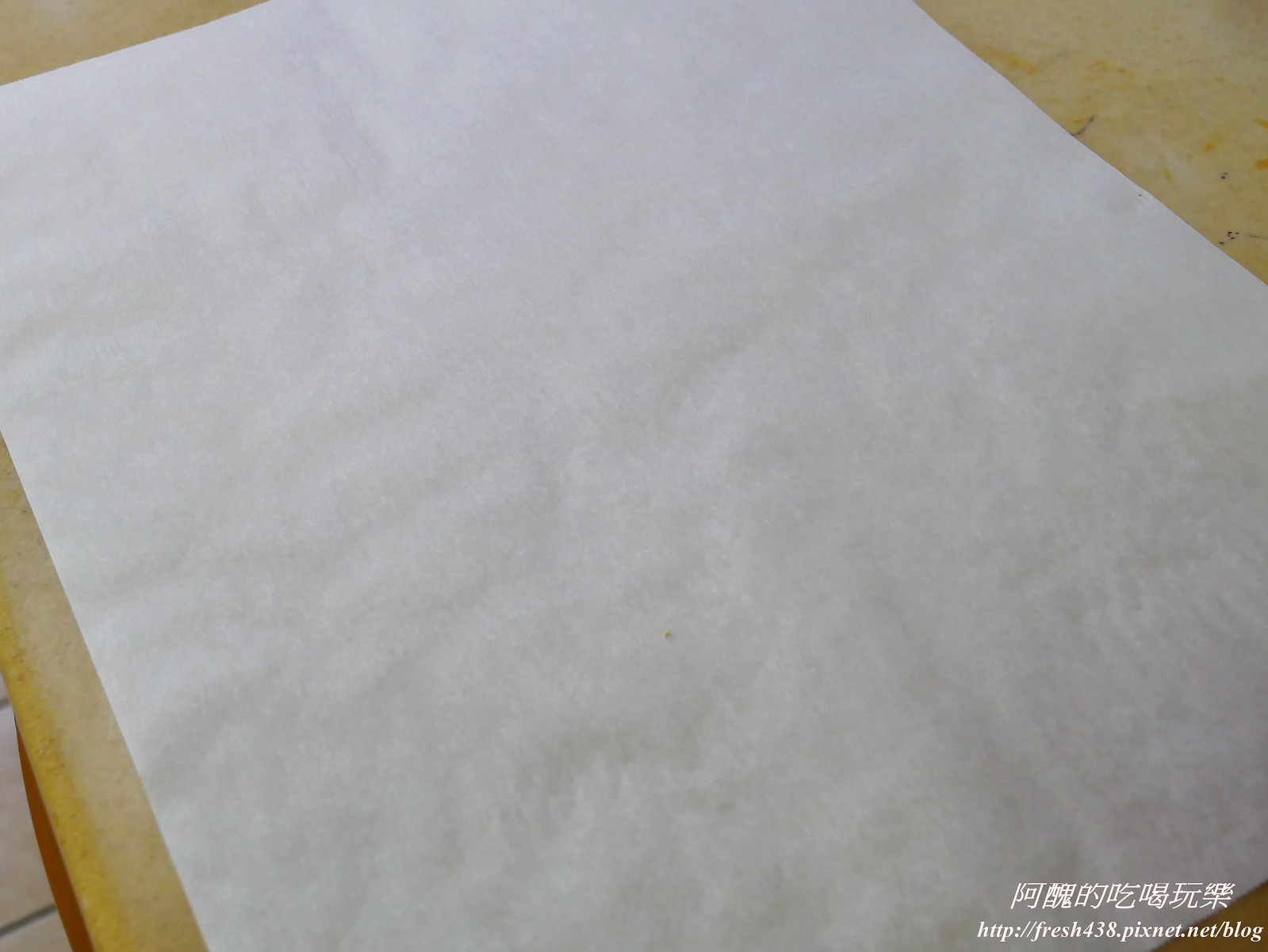The image shows a perfectly laid-out sheet of white paper or possibly parchment, placed at an angle on a yellow table or countertop, with its top near the top left and its bottom near the bottom right of the frame. The table appears to have a slightly darker yellow edge on the left side. The scene includes part of a red item visible below the table, resting on a floor made of white ceramic tiles. The paper is completely blank with a slight crinkling near the bottom, and the table surface may have a speckled effect, suggesting a countertop. In the bottom right corner of the image, a watermark reading "fresh438.pixnet.net/blog" is visible, accompanied by some Asian characters, likely Chinese, Japanese, or Korean.